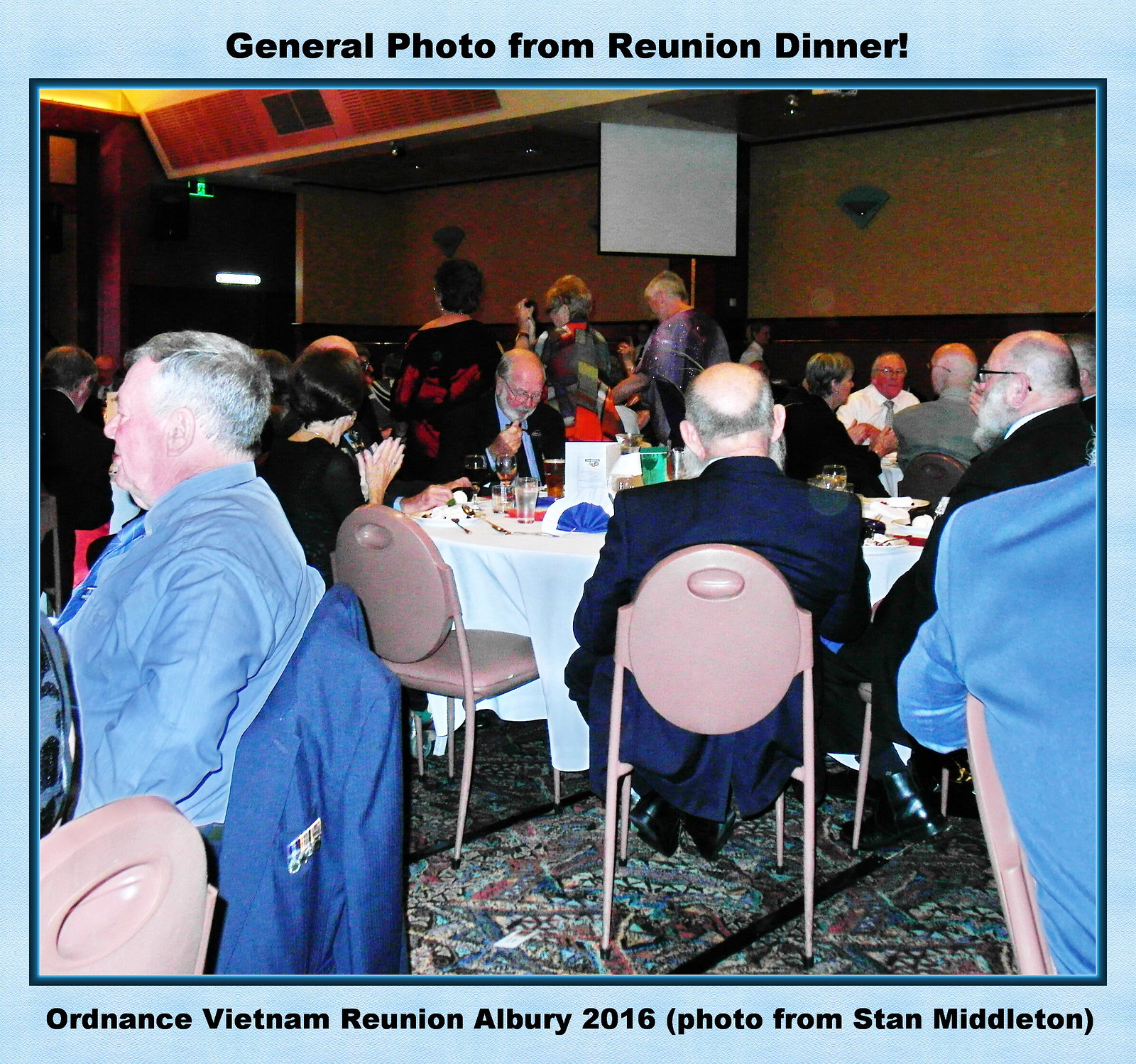The photograph captures a bustling reunion dinner event hosted in a spacious, carpeted banquet hall, featuring a sea of round tables draped in white tablecloths and surrounded by a mix of beige and pink chairs with circular backrests. Predominantly attended by elderly individuals—most men sporting white, gray, or balding heads, and women with either dyed, white, or gray hair—the guests appear to be in their 60s and 70s or older. The men are dressed in suit jackets paired with nice shirts, while the women are in elegant dresses or pantsuits with coats. There’s an air of camaraderie as people sit around tables, some enjoying wine, while a few others stand and converse in the background. A notable detail is a blue-shirted man with his blue jacket draped over his chair, showcasing medals. The room is adorned with a carpet with an intricate pattern. The image is enclosed in a light blue border, with text at the top that reads "General Photo from Reunion Dinner" and additional text at the bottom declaring "Ordinance Vietnam Reunion Albury 2016," attributed to Stan Middleton. Prominent in the layout is the back of a gentleman's head, capturing a moment of reflective dialogue or merriment among the attendees.